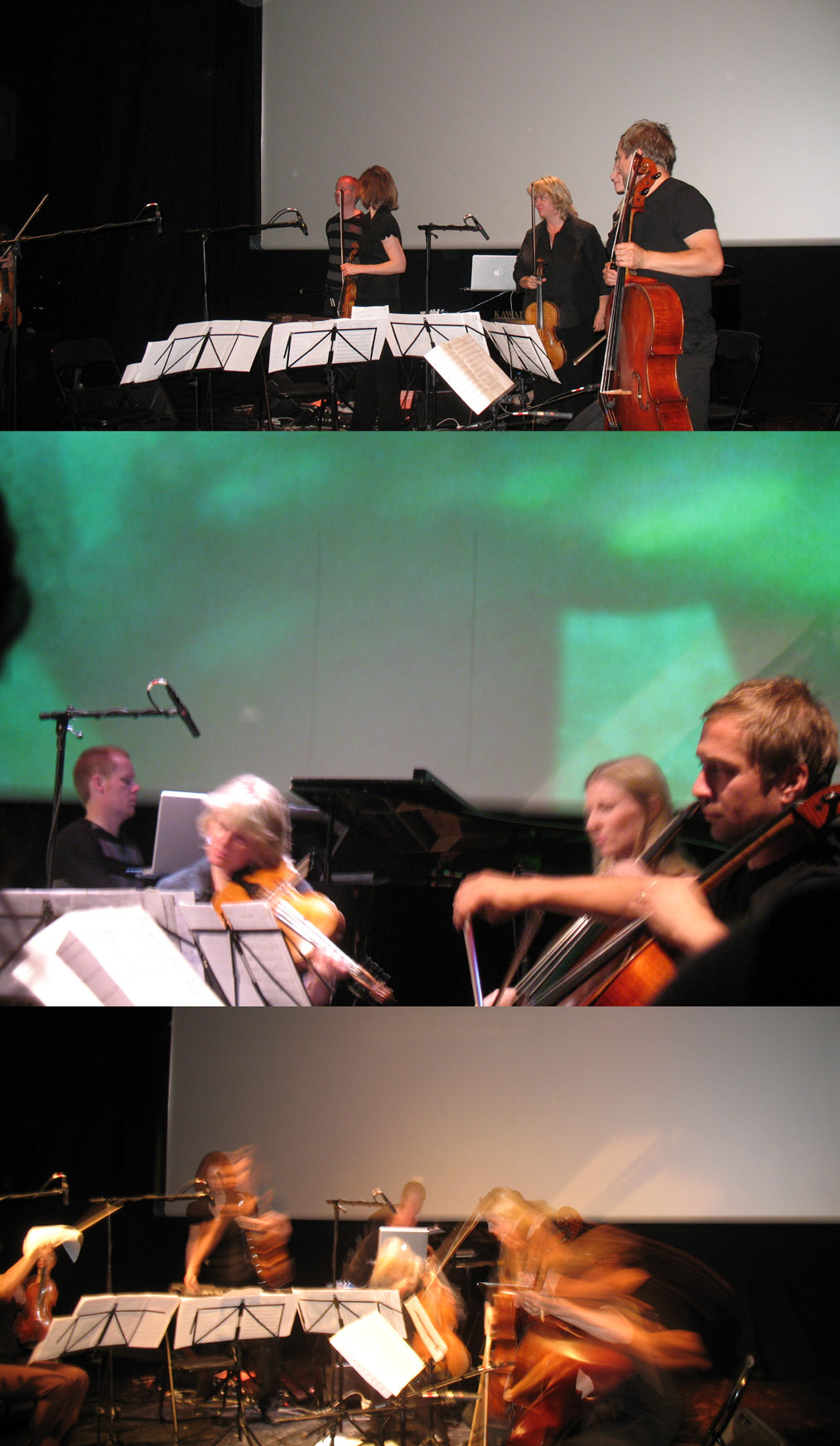A series of three rectangular photographs captures a live orchestral performance on stage. The central photograph is slightly taller in height and showcases a group of four musicians. Two of them are dressed in short-sleeved black outfits, one in a long-sleeved black outfit, and a fourth person on the left in a striped black and brown shirt holding a violin while looking backwards. The person in the middle, who has blonde hair, is playing a violin or viola, and another musician on the right is with an upright bass. However, indicating the changing layout, the central part also presents four musicians seated while performing, suggesting the instrument held might be a cello given the upright posture. The stage is adorned with music stands filled with sheet music, and a Mac laptop can be seen. The upper photograph highlights these same musicians and their instruments, while the lower photograph is notably blurry, capturing the motion of the performance, potentially due to the rapid movements of playing instruments like the violin. A green light casts an intriguing hue over the scene from an unspecified source, adding a unique atmosphere to the visuals.